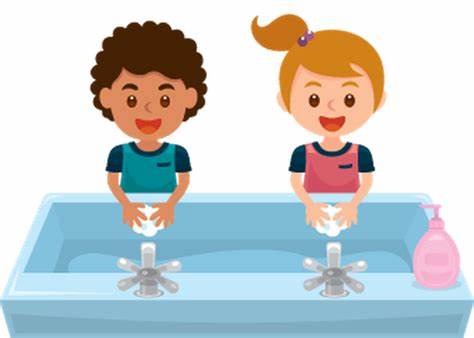This colorful cartoon image features two children standing at a large rectangular sink with two faucets, diligently washing their hands. The sink is blue with silver handles and is equipped with a pink soap dispenser located on the right side. To the left stands a smiling boy with tan skin, short curly brown hair, and brown eyes. He is wearing a teal or green shirt and has soap suds on his hands. On the right is a smiling girl with pale skin, blonde hair tied into a ponytail with a purple hair tie, and brown eyes. She is wearing a red shirt and also has soap bubbles on her hands. Both children are happily engaged in washing their hands, with water visible in the sink.